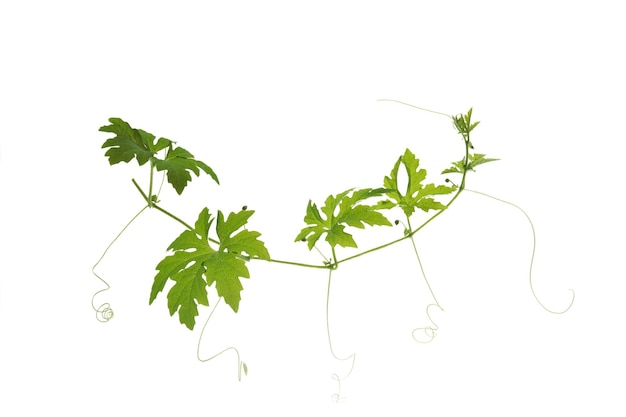This image showcases a green vine set against a clean, white background, which emphasizes its natural details in a minimalistic and scientific manner. The vine, which features several clumps of leaves connected to a thin stem, curves upward on the left and right sides. The leaves vary in size and shape, with the leftmost leaf appearing darker green while the others are lighter, likely indicating younger leaves. Additionally, delicate, thread-like tendrils emerge from the stem, curling into small, corkscrew shapes. This professionally lit photograph captures the intricate details of the vine, highlighting its structure and the positioning of its leaves and tendrils.